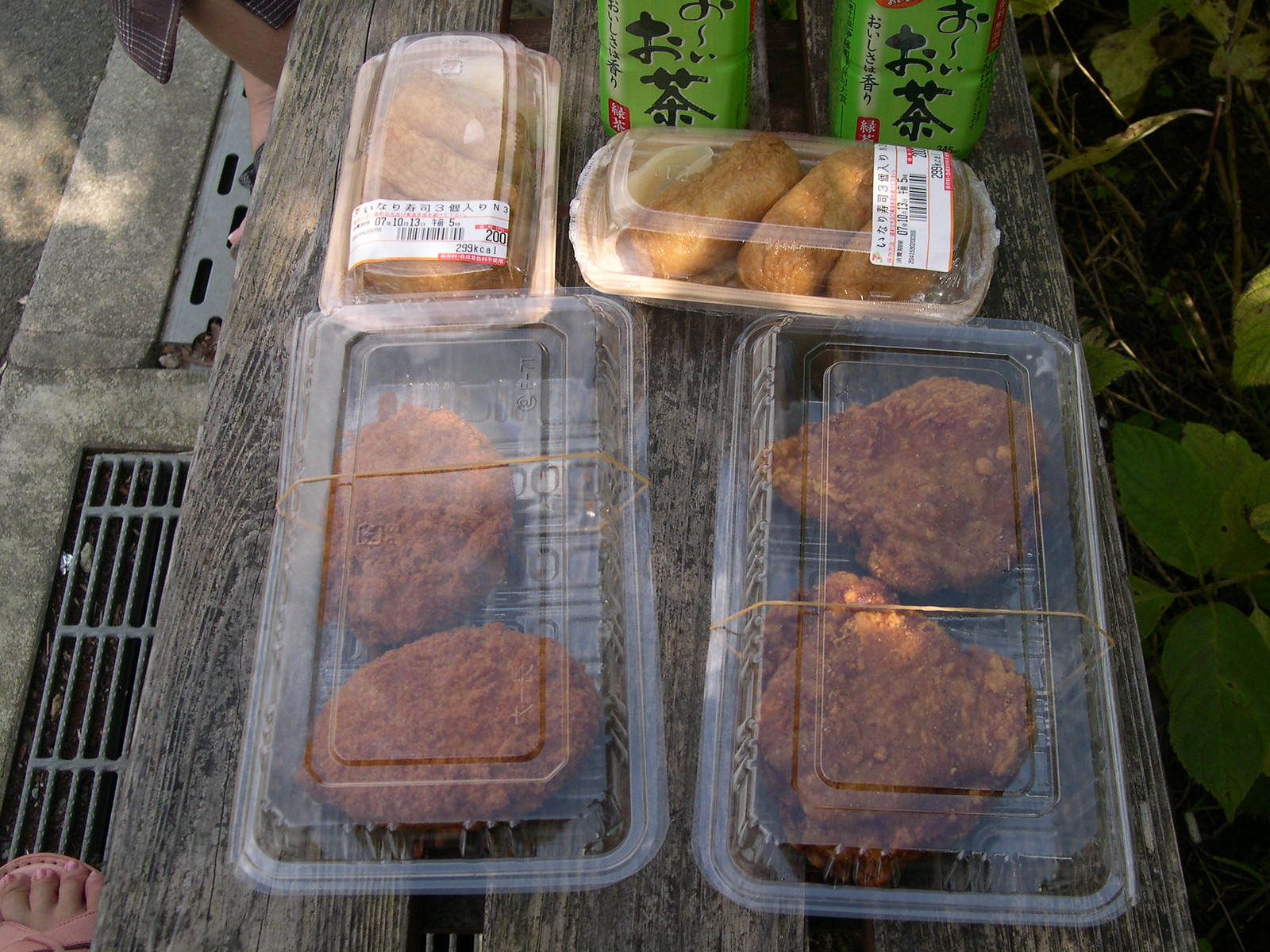An overhead view captures a brown park bench composed of three slats sitting beneath various food containers. The middle bench slat runs vertically through the center of the image, with two additional slats flanking it on either side. In the lower left, a fair-skinned foot with pink toenail polish peeks in, wearing pink flip-flops, standing on a grate designed for water drainage, bordered by concrete. Above this, the edge of a skirt and a leg are visible. Along the right edge, an inch-and-a-half strip of green leaves frames the scene.

The bench holds four transparent plastic containers of food. At the bottom, a long rectangular container with two round brown patties secured by a rubber band stands vertically. To its right lies an identical container with two well-cooked chicken breasts. Above these, a smaller rectangular container positioned horizontally holds three golden-brown egg rolls. At the top center, another container contains light brown potato wedges, each labeled with a white sticker. Topping off the arrangement, two green cans of soda with black Chinese writing nestle above the egg roll container.